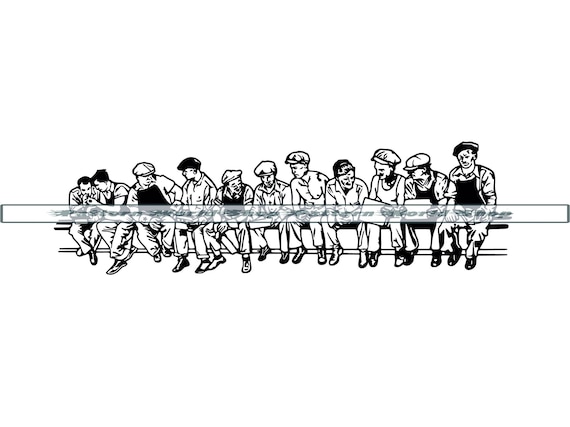This artwork, displayed against a pristine white background, is a monochromatic drawing rendered entirely in black and white. It portrays a group of men dressed in vintage, blue-collar worker or factory worker attire, evocative of a bygone era. The men are seated in a row, exuding a sense of camaraderie and collective perseverance. Encircling the group is a transparent white bar featuring text, adding an additional layer of context or narrative to the composition. The juxtaposition of the stark white background with the intricate details of the workers' attire and expressions draws the viewer’s attention to the subjects, emphasizing their historical and cultural significance.